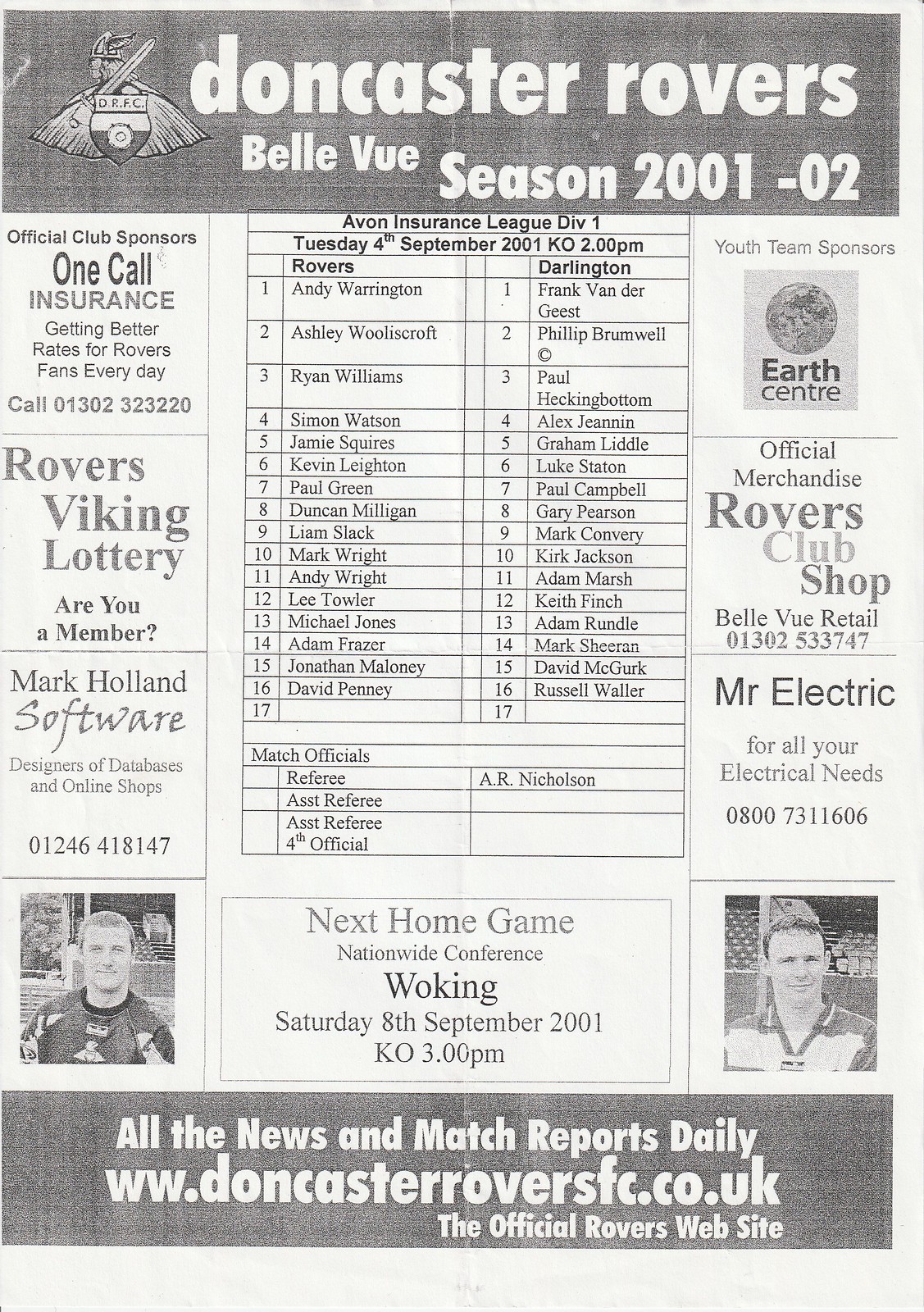The image is a black and white page from a Doncaster Rovers soccer program for the Bellevue season 2001-02. At the very top, it prominently reads "Doncaster Rovers Bellevue season 2001-02" with the Doncaster Rovers' Viking insignia to the top left, depicting a Viking holding a sword and shield facing left. Below, the page features several sections and advertisements:

- The left column highlights the official club sponsors, "One Call Insurance," promising better rates for Rover fans, followed by ads for the "Rover Viking Lottery" and "Mark Holland software designers." There are also images of soccer players near the bottom.
- The right column includes youth team sponsors "Earth Center," "official merchandise from the Rovers Club Shop at Bellevue Retail," and an ad for "Mr. Electric for all your electric needs," along with player images.

At the center, a significant portion is dedicated to a match scheduled in the "Avon Insurance League Division 1," set for Tuesday, 4th September 2001, with a kickoff at 2:00 p.m. This section features a data table listing the players from "Rovers" on the left and "Darlington" on the right, alongside match officials including the referee and assistant referees.

Towards the bottom, there is an ad for the next home game in the "Nationwide Conference" against Woking on Saturday, 8th September 2001, with a kickoff at 3:00 p.m. Finally, a banner across the bottom reads "All the news and match reports daily at www.doncasterroversfc.co.uk – the official Rovers website."